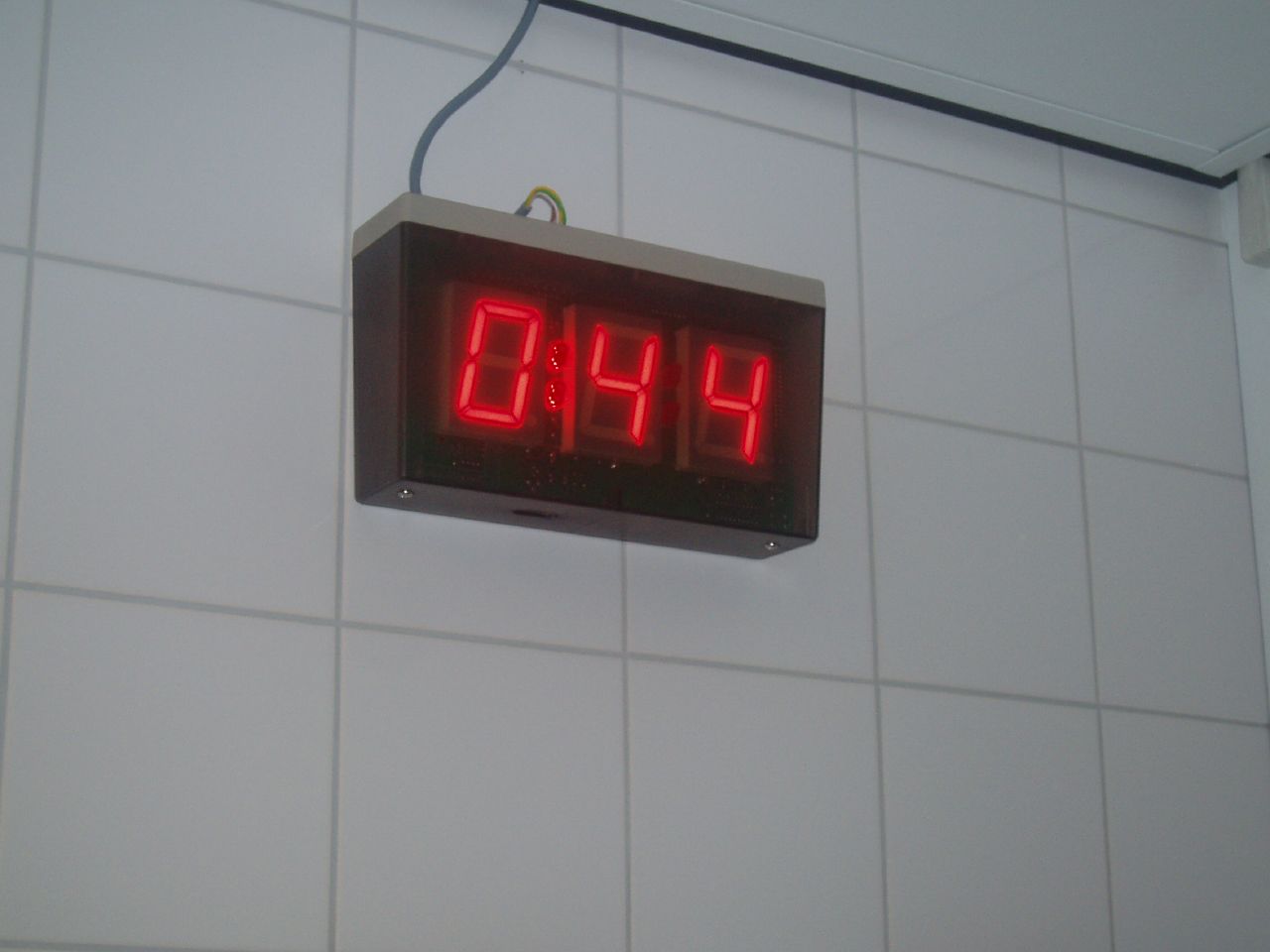The image features a vintage timer mounted on a pristine white wall composed of small, glossy square tiles with clean white grout, evoking the feel of a bathroom or perhaps a sterile laboratory environment. The timer itself is a large, rectangular black box displaying an LED readout of "0:44" in red digits, suggesting seconds remaining. A wire extends from the top of the timer and runs straight up toward the ceiling. The seamless cleanliness and the stark, almost clinical setting of the tiled wall contribute to a sense of isolation or controlled environment, while the mysterious context of the timer adds an element of intrigue.